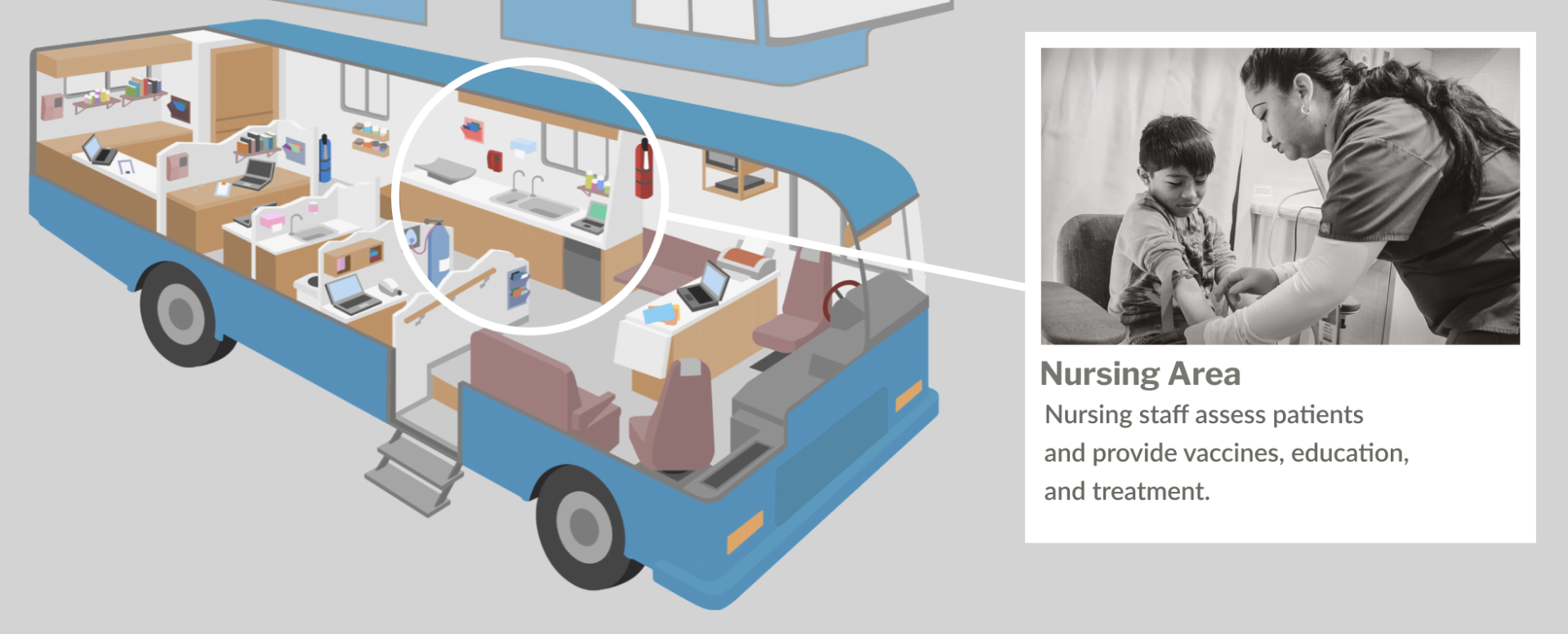The image depicts a mobile clinic, designed as a bus with a transparent cutaway view revealing its interior. The vehicle, which is light to medium blue, is equipped to provide comprehensive healthcare services at various locations. The bus features a drop-down step for easy access. Inside, the clinic is fully outfitted with a sanitation sink, numerous desks with computers for patient check-in, and designated areas for various medical procedures such as vaccinations.

Prominently displayed in the image is a photograph in black and white labeled "Nursing Area." This section shows a female nurse administering a vaccine to a young boy seated in a brown chair. The nurse, with her hair tied back in a ponytail, is wearing small gold hoop earrings and a dark-colored shirt. The boy, who has short hair, has rolled up the sleeve of his long-sleeved shirt to receive the injection. Both the nurse and the child appear to be of Central American descent. The accompanying text explains that the nursing staff assesses patients and provides vaccines, education, and treatment.

Overall, the mobile clinic is depicted as a versatile and well-equipped medical facility akin to a traditional clinic, highlighting its capacity to deliver essential healthcare services efficiently.